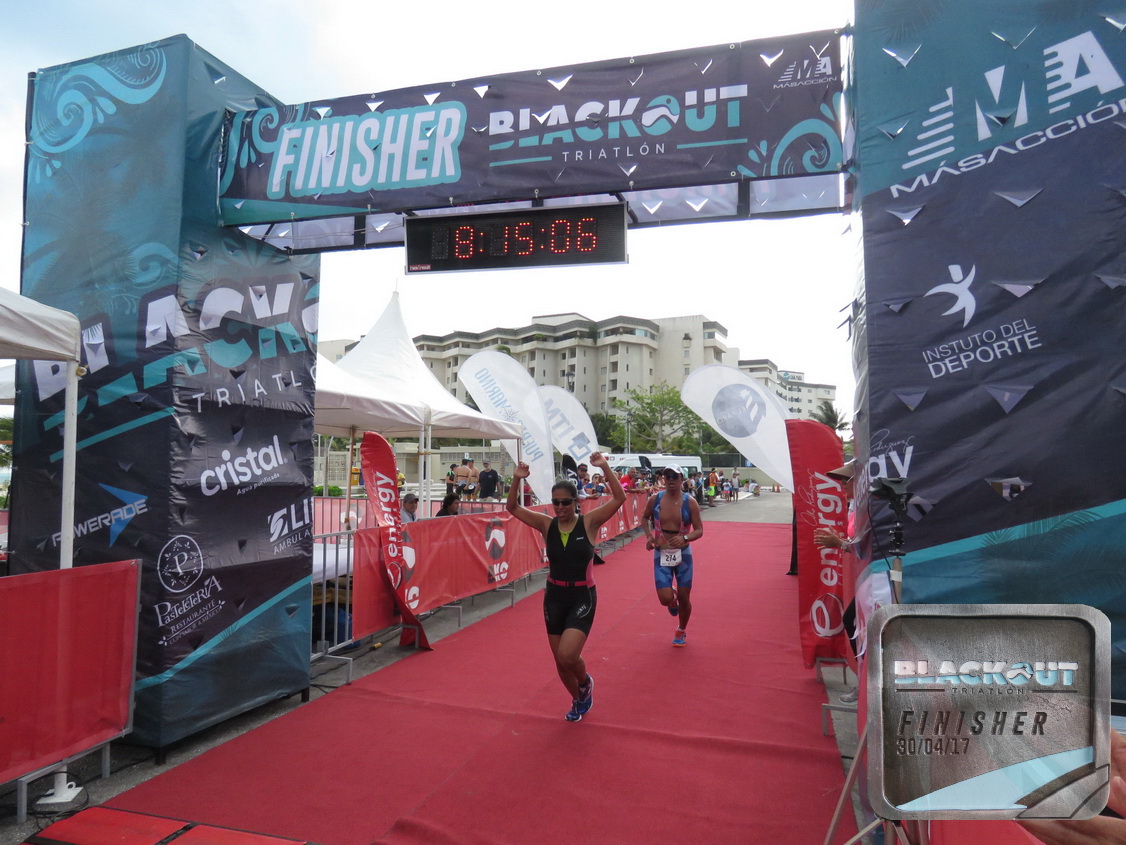This image captures the intense moment at the finish line of the Blackout Triathlon. Leading the race is a middle-aged woman dressed in a black outfit—black shirt and black shorts—crossing the finish line with her arms raised in triumph. Behind her is another runner, a young man wearing blue shorts, a blue unzipped bodysuit, and a white hat. They are both running through a fenced area adorned with red carpeting. Above them, a digital clock displays the finish time as "8:15:06," encapsulated within an arch that reads "Finisher Blackout Triathlon" in white font. The backdrop features large apartment buildings and is dotted with various energy signs, advertisements, white tents, and a gathered crowd of spectators lining up along the edges, eagerly watching the runners complete their race. The overcast sky adds to the dramatic atmosphere of the scene.